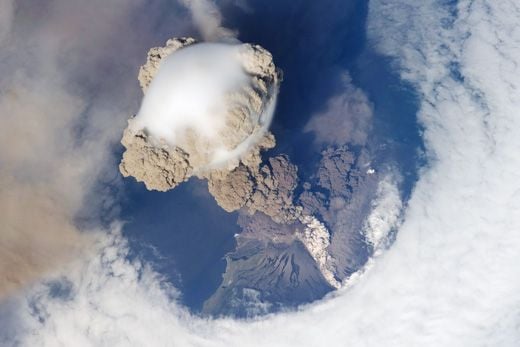This aerial image, taken from a high vantage point, possibly from a plane or drone, captures the dramatic aftermath of a volcanic eruption. Dominating the center is a towering mushroom cloud of ash, billowing intricately with swirls of both stark white and light brown. Encircling this colossal plume is a ring of wispy clouds that extend from the top right to the bottom right, curving almost to the left edge. The base of the plume reveals a darker brown stem-like formation that appears to trail down into the central dark area, which could be the opening of the volcano itself. Surrounding the core eruption are muted, blurred gray-brown rocky landmasses, contributing to the landscape’s rugged texture. At the periphery, deep blue tones, suggestive of the ocean or possibly a vast expanse of sky, frame the scene, contrasting vividly with the chaotic central ash cloud.